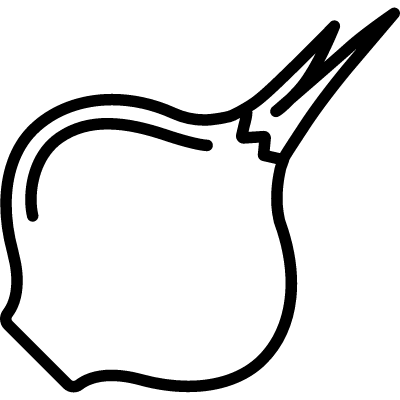This image is a simple black-and-white illustration resembling a sprouted onion, presented in a minimalist style. The illustration features a bold black outline against a plain white background. The onion-shaped figure is oriented diagonally from the lower left to the upper right. Its base is flat and positioned at the lower-left corner, while the bulb is rounded, tapering to a point from which two sprouted stems extend, forming a V-shape that reaches towards the upper right. Inside the bulb, there is a curved line following its contour, adding a sense of dimension, and a zigzag line where the pointed sprouts emerge. The entire image is devoid of any texture or color, emphasizing its clean, clip-art-like simplicity.